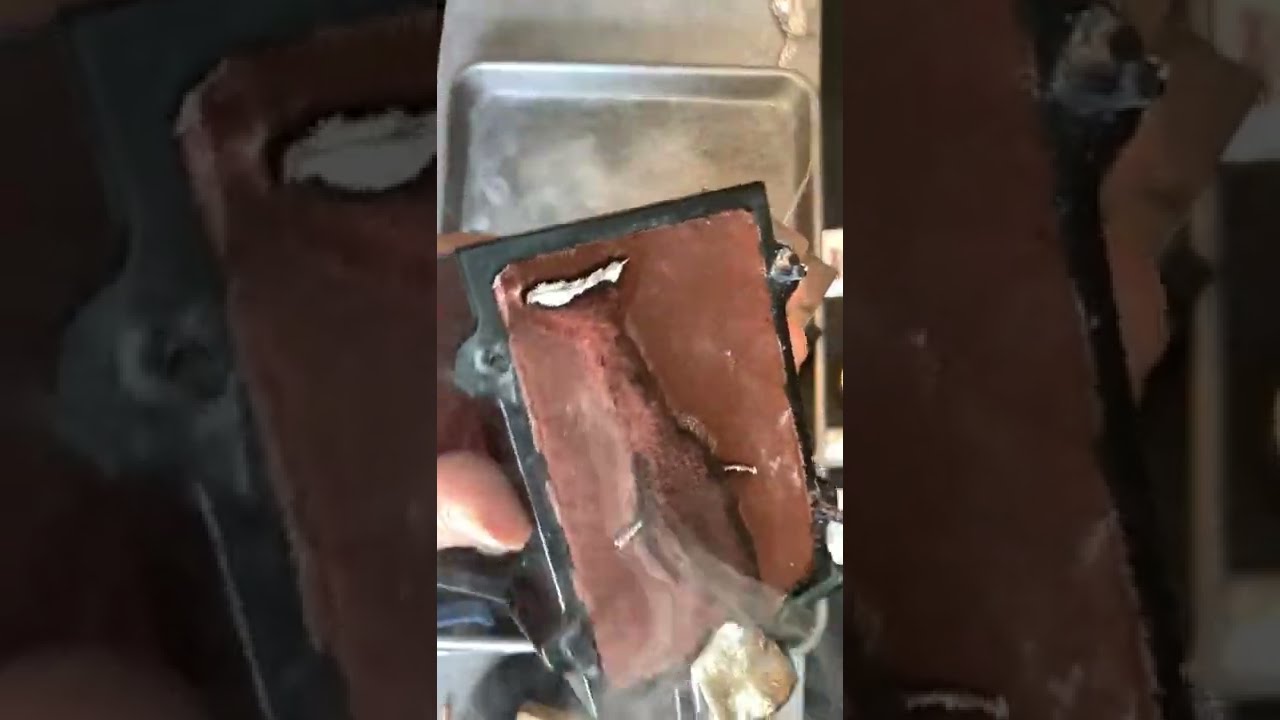The image features a top-down view of a black rectangular case being held by a person's hand, including their thumb and a portion of their knuckle, over a silver rectangular tray that rests on a silverish-gray countertop. The case encloses a terracotta-brown object with an intricate pattern resembling a fossil, complete with a feather-like indentation or design in the center. This pattern includes white lines, one thicker line near the "tail," and possibly represents an abstract or random shape. The entire scene is slightly blurry, with parts of the case covered by a thin film. Additionally, the entire image is framed within a portrait orientation and is surrounded on the left and right by zoomed-in and dimmed views of the object, creating a cohesive and detailed visual composition.